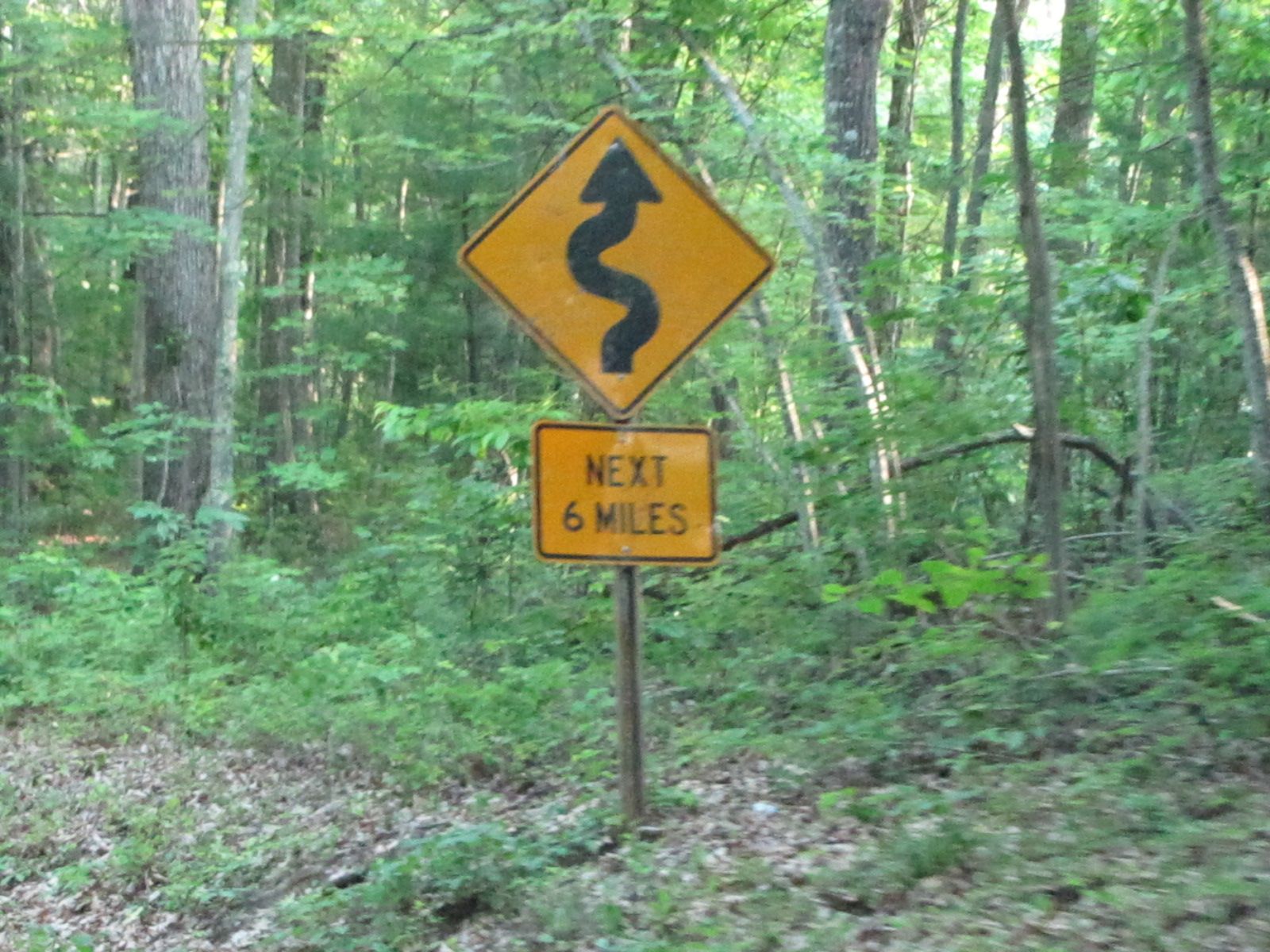In this color photograph, we observe a tranquil wooded area. At the very bottom of the image, patches of bare ground are interspersed with small bursts of green vegetation, accompanied by numerous fallen twigs indicative of previous seasons or wind. The backdrop is dominated by the forest, characterized by a dense assembly of tree trunks in varying shades of dark and medium gray, which blend with the similarly muted tones of the leaves. The subdued and almost desaturated colors suggest the use of a filter or special effects, which soften what would otherwise be the vibrant greens of nature.

Prominently situated in the center of the frame is a road sign mounted on a steel pole. The top sign is yellow, arranged in a diamond shape, and features a black squiggly line with an arrow, signaling an upcoming winding road. Just below this warning, a smaller sign declares that the curvy stretch extends for the next six miles. The overall composition is serene yet subtly dynamic, capturing the essence of a quiet forest scene intersected by a cautionary symbol of human navigation.